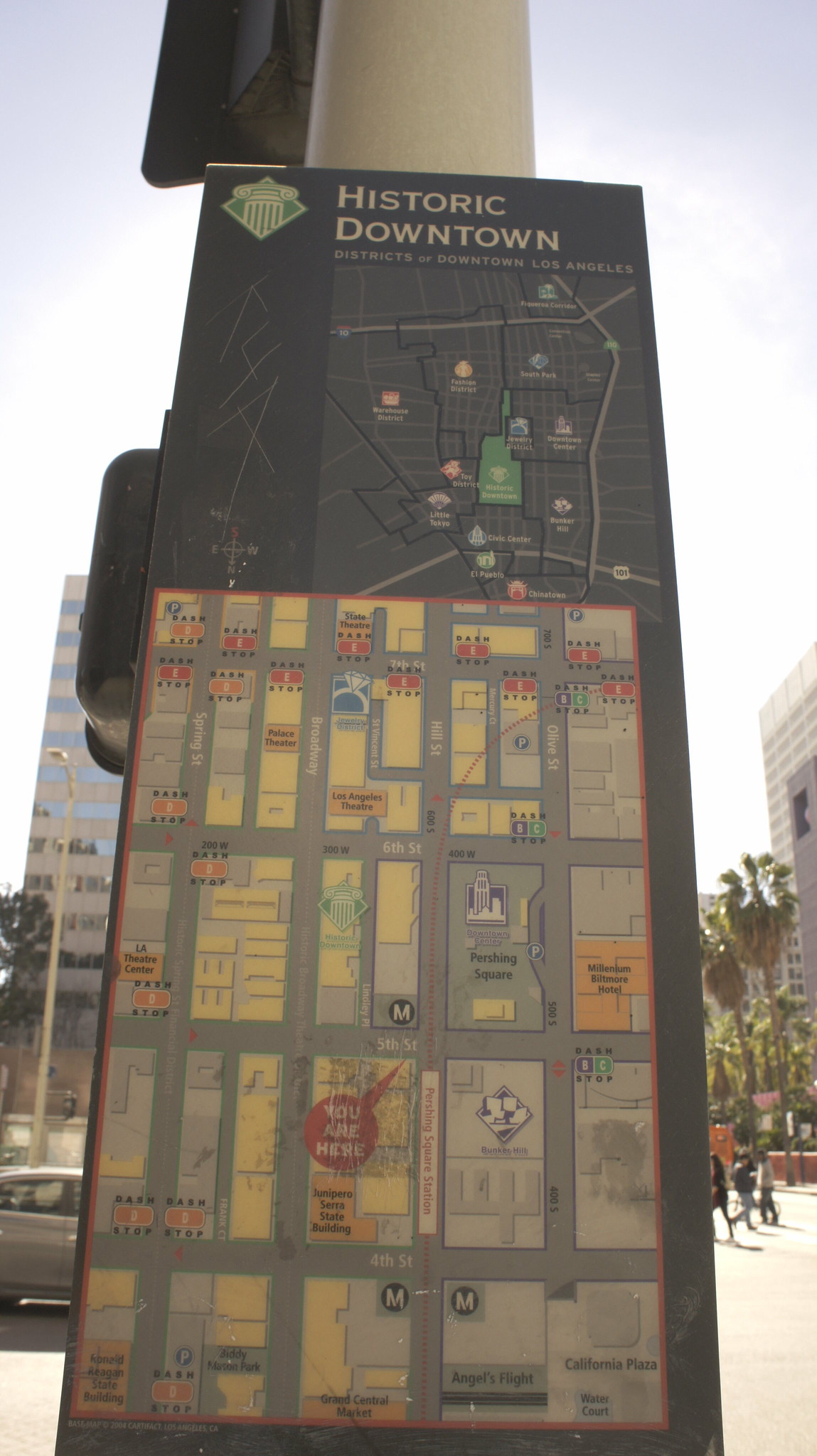This image depicts a detailed road map primarily rendered in black, resembling a board. At the top of the map, a distinctive diamond-shaped symbol is present. On the right side, "Historic Downtown" is clearly written. The map includes both black-and-white and colored segments, featuring roads represented by black and grey lines, as well as various icons and routes marked in green, red, and blue.

In the bottom left corner, there is a larger, zoomed-in section of the map. This section is distinguished by long, yellow rectangles through which roads traverse. Notably, the fourth line of these rectangles contains red text and an arrow pointing to a corner with the indication "You Are Here."

Additional details on the map show various colors, including orange writings and prominent red icons, although the absence of a map key means the symbols' specific meanings are unclear.